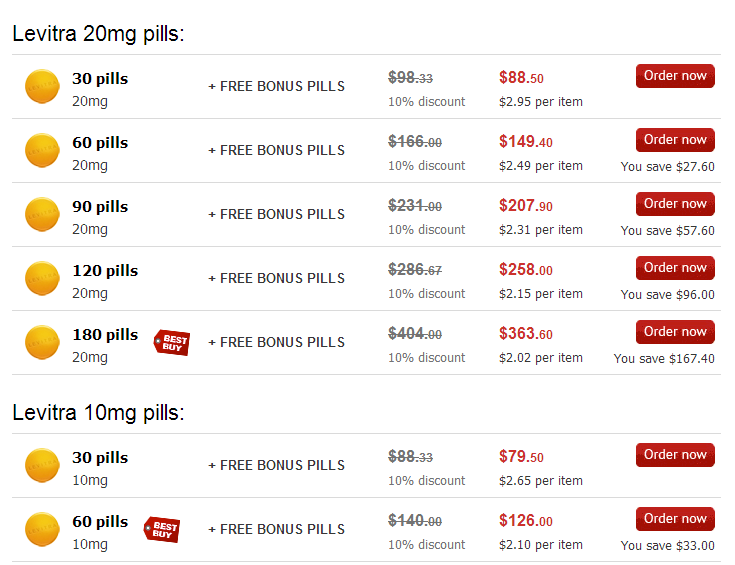An assortment of Levitra tablets in various dosages and quantities is available for purchase. Options include 20 mg pills in counts of 30, 60, 90, 120, and 180, as well as 10 mg pills in counts of 30 and 60. With each purchase, free bonus pills are included to enhance value. Price savings are substantial: save $27.60 on select options, up to $167.40 on larger quantities. Order now to benefit from these significant discounts and offers.